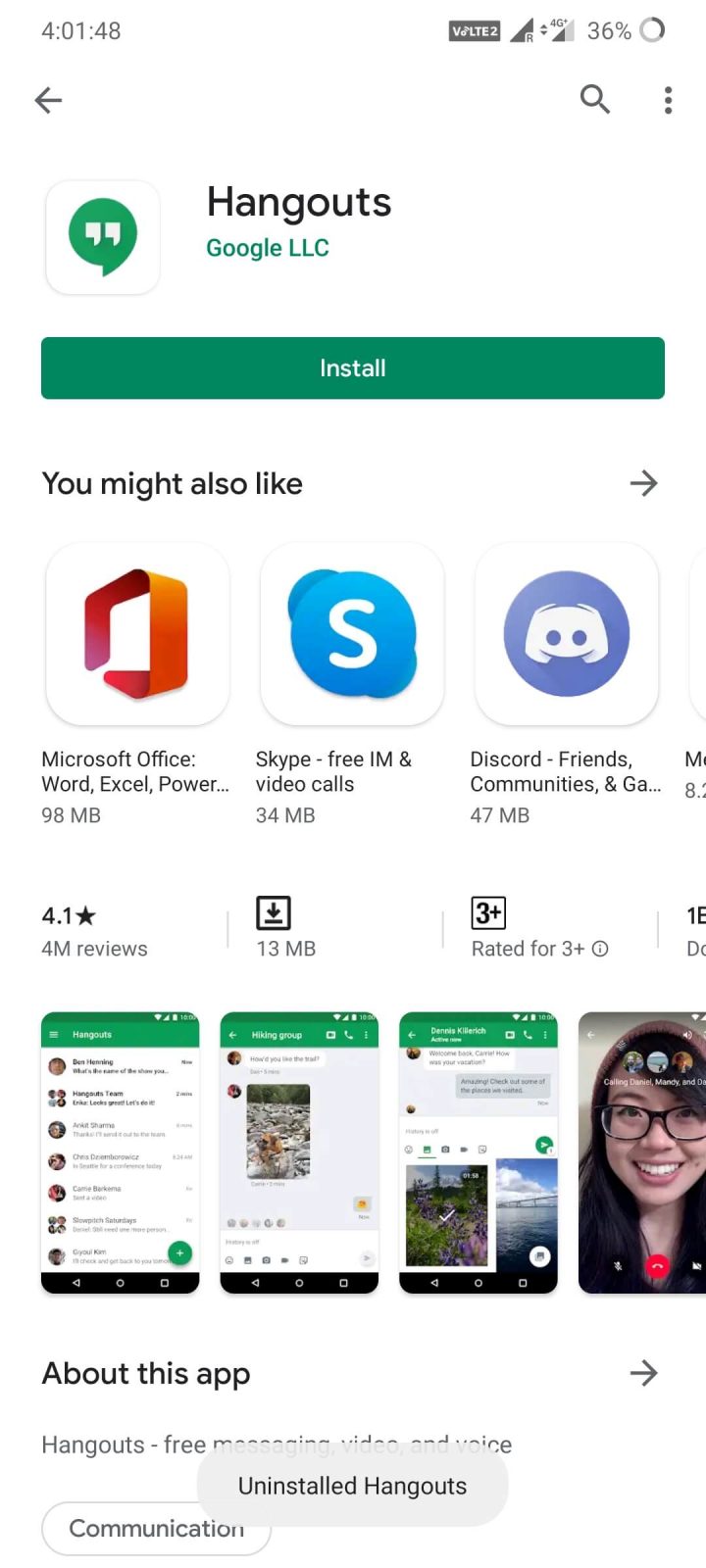A smartphone screen displaying the Google Play Store is shown. The status bar at the top indicates the time as 4:01:48, with icons on the right side for a 36% battery level, dual SIM, roaming, and 4G LTE connections.

Prominently featured in the Play Store is the Hangout app by Koji LLC. The app's icon is a green conversation bubble against a white background. Below the icon is a green "Install" button. Further down, a recommendation section suggests other apps like Microsoft Office (orange and red icon), Skype (blue and white icon), and Discord (dark blue and white icon).

The Hangout app is rated 4.1 stars, has 4 million reviews, and is 13 MB in size. It is suitable for users aged 3 and above. The description includes images of the app and states, "Hangout - free messaging, video, and voice."

At the bottom of the screen, a pop-up notification reads "Uninstalled Hangout," indicating that the app has been successfully uninstalled.